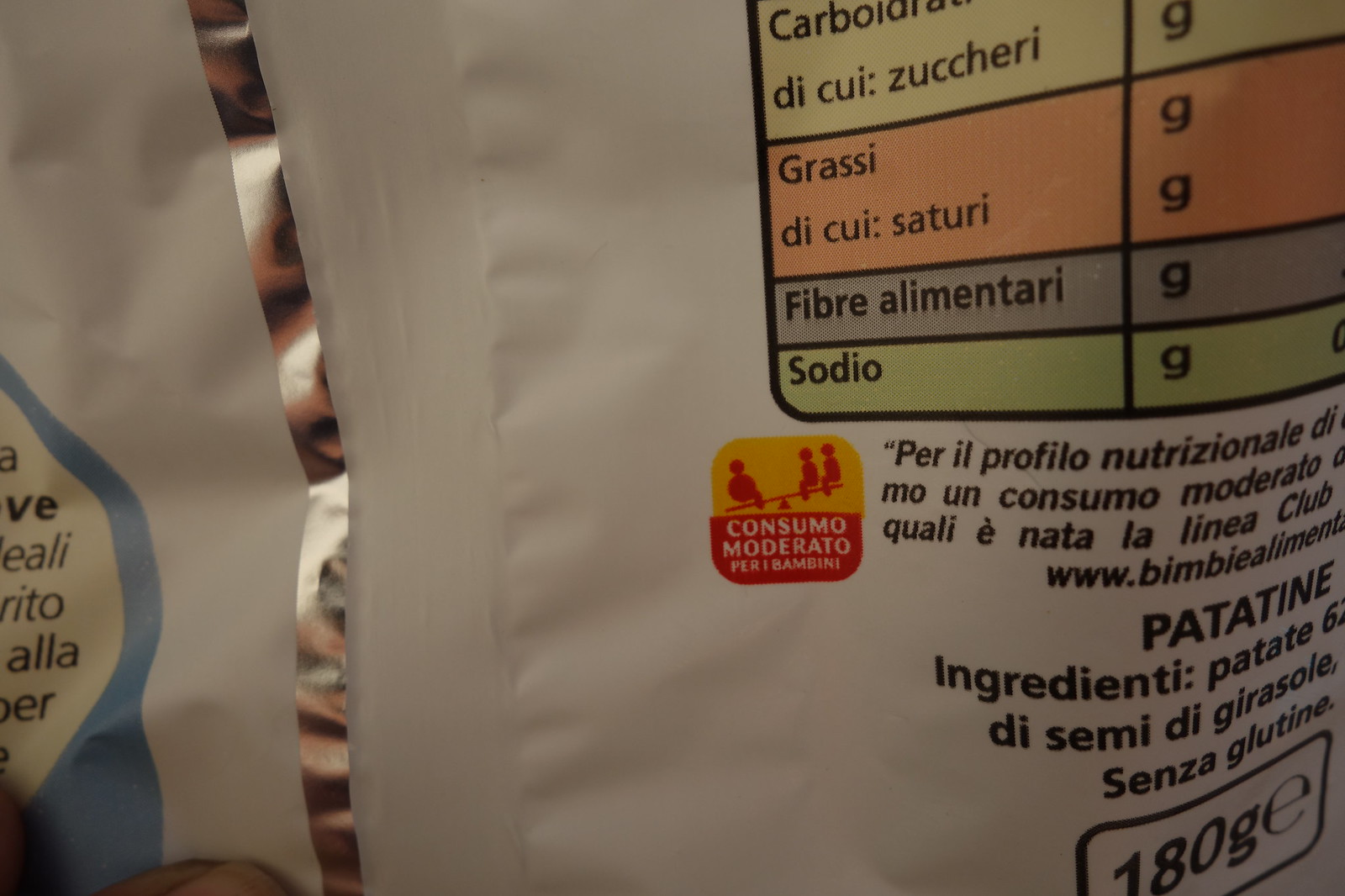This photograph, taken with a high-resolution camera, depicts a product packaging with visible text primarily on the bottom-left corner. The text is in a foreign language and includes several sections, each highlighted in different colors. The sections and their respective colors are: "Grassy" (Red), "Fiber" (Blue), "Sodio" (Green). Additionally, there is text that reads "Dikui: Saturi" and "Alimentary." The package's nutritional information lists the weight as 180 grams. Although the details are somewhat unclear, the image is captured against a white background.